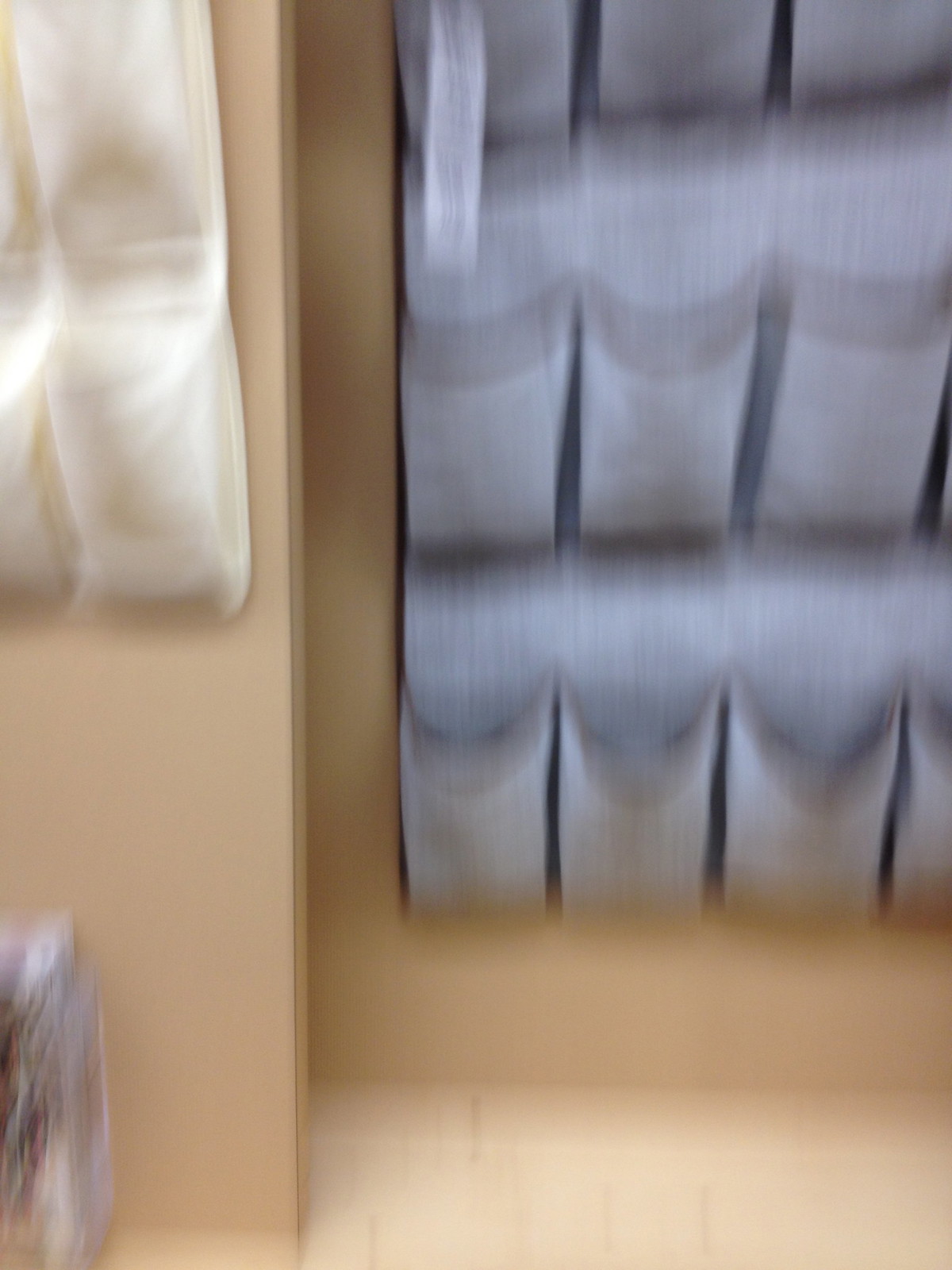The photograph, though incredibly blurry and taken with vertical motion, seems to depict an interior setting, possibly inside a store or a specific room such as a mailroom or bathroom. The image features a tan-colored wall that forms a corner with another recessed wall, creating a shadowed area on the right side. The recessed wall is adorned with a gray fabric organizer containing individual pockets arranged in three visible rows, each row having three to four pockets wide, potentially used for shoes or toiletries. On the left side of the main wall, there is a partially visible white fabric organizer with at least two pockets wide and two pockets high. The floor beneath appears to be tiled in a tan color, and there seems to be a box or trash can positioned near the front wall, which also has white pouches attached to it. The photograph's overall clarity is compromised, making fine details hard to discern.